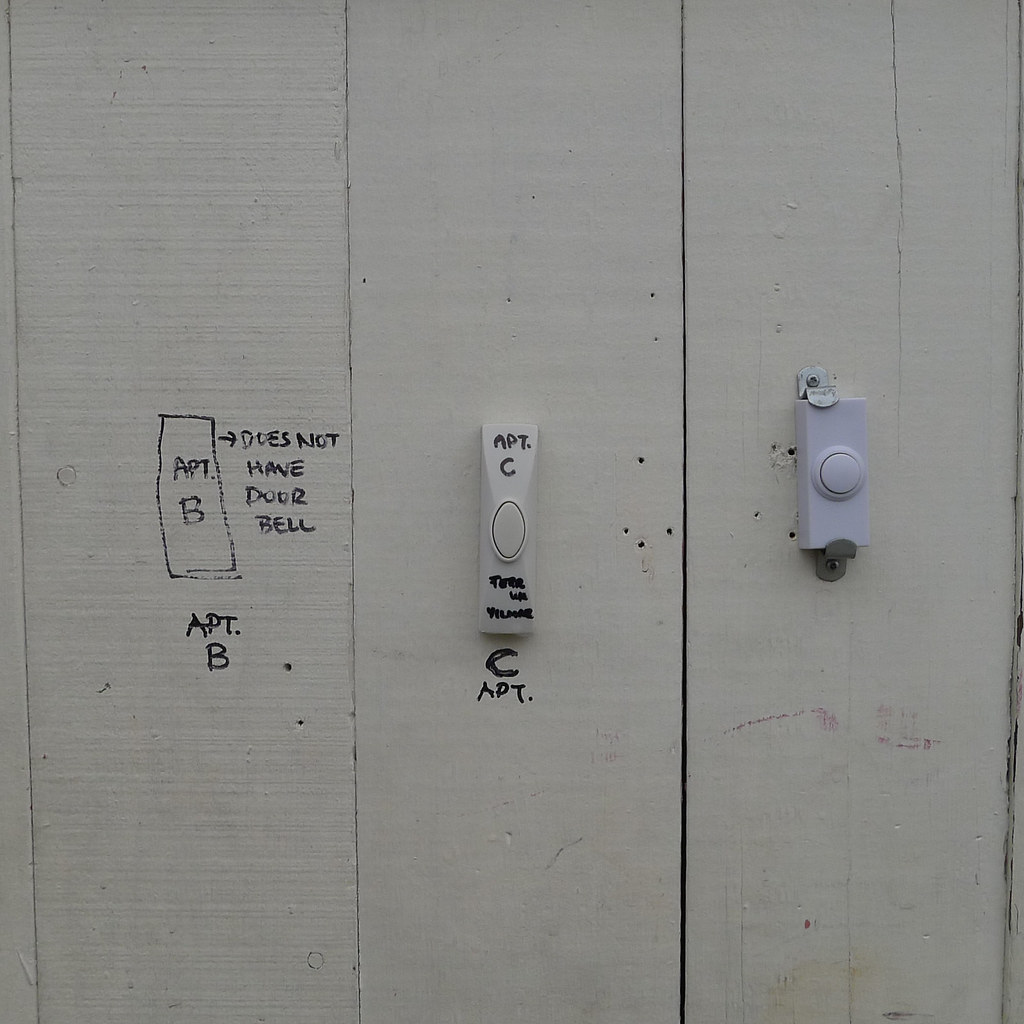In this photograph, a dimly-lit, white-painted wooden wall is divided into three vertical panels, each featuring doorbell-related information. The center panel showcases a white doorbell button with "Apartment C" written in black marker both above and below the button. Additional illegible text is noted at the bottom of the button. The right panel displays another white doorbell, more modern in design, with a rectangular shape and a circular button in the center, though it lacks any textual labeling. The left panel, in contrast, features a hand-drawn rectangle intended to represent a doorbell. Inside this rectangle, "Apartment B" is inscribed in black marker, with an additional note "does not have doorbell," emphasizing the absence of a functioning doorbell for Apartment B. The concise directional and informational notes provide clear guidance regarding the presence and absence of doorbells for these apartments.